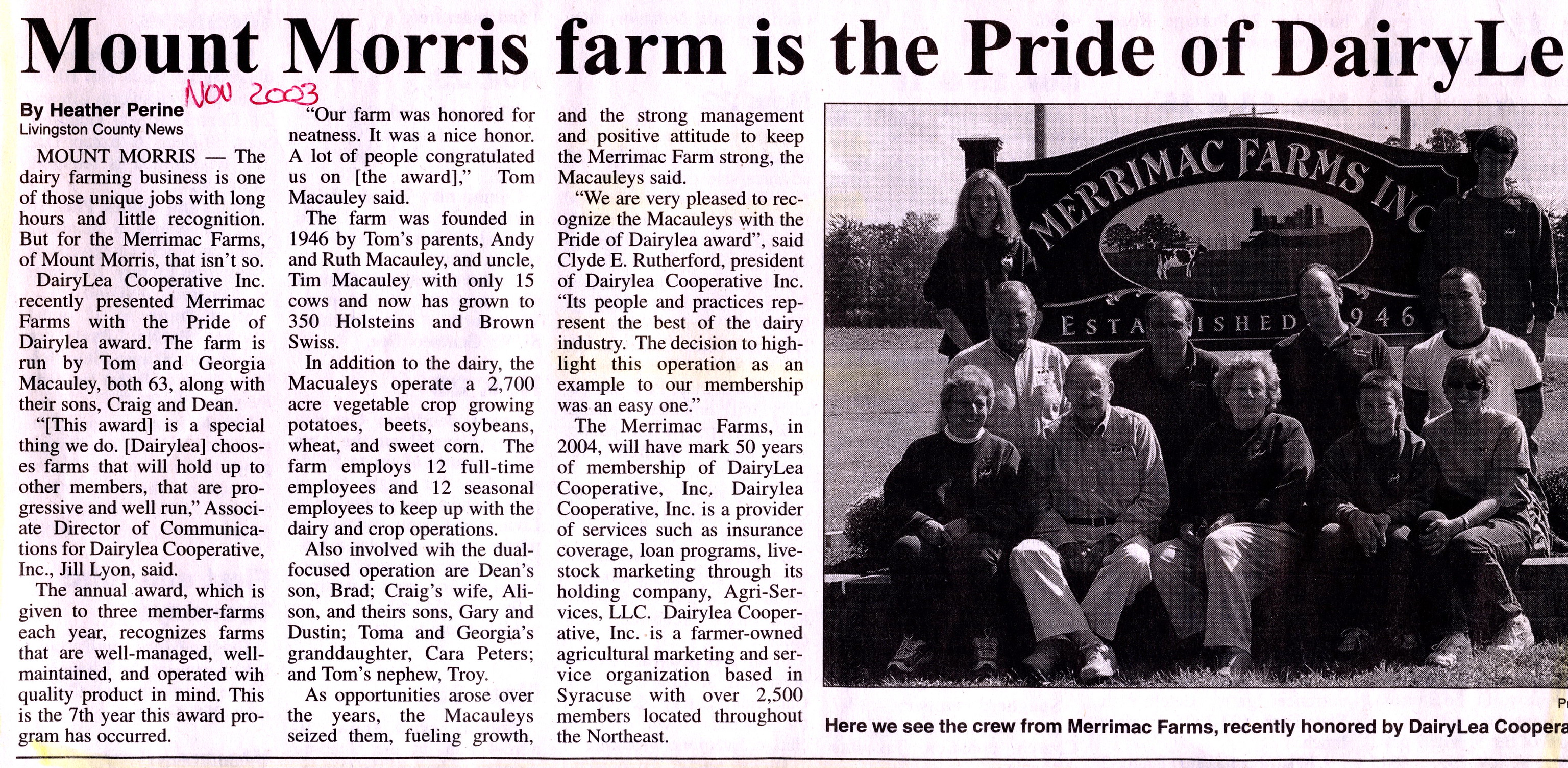This newspaper clipping features a headline that reads, "Mount Morris Farm is the Pride of Derry Lee," although the headline is truncated. Authored by Heather Perrine, identified in the byline from the Livingston County News, the article spans three columns of text on the left side, detailing the accomplishments of Mount Morris Farm. A handwritten note in red ink, "November 2003," is visible near the byline. To the right of the article, there is a photograph of a diverse group of individuals, ranging in age from elderly men to a young boy around twelve, all posing in front of a sign that reads, "Merrimack Farms Inc., Established 1946." The caption below the photo states, "Here we see the crew from Merrimack Farms recently honored by Derry Lee," though it is also partially cut off. The image also shows yellow highlighter marks, which appear to be bleed-through from another page originally placed on top of this one.